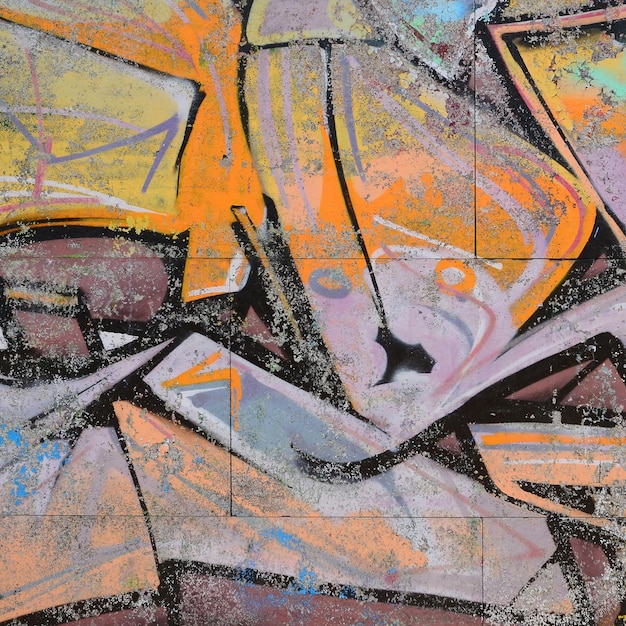This close-up photograph captures an abstract piece of street art on what appears to be a cinder block wall, characterized by the visible seams between the bricks. The artwork is a vibrant mix of colors including bright oranges, yellows, pastel blues, pinks, and occasional muted grays, with black lines interspersed throughout. The graffiti resembles fragmented, weathered text that might depict a frightened figure looking over their shoulder, though the interpretation is ambiguous. The paint has chipped in various places, unveiling the underlying stone and adding to the textured, aged appearance of the composition.